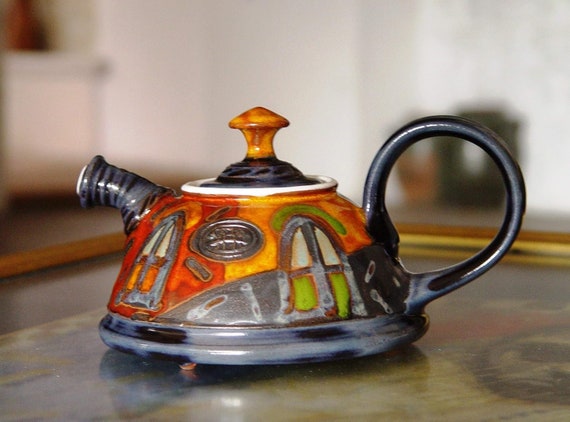This detailed photograph features a striking, colorful teapot situated on a flat surface, resembling a grill often seen in Japanese cuisine like at Benihana. The teapot boasts a large black handle arching from its body and a short, gray spout adorned with black stripes extending from the left. Its body comprises an array of vivid colors, including red, yellow, lime, black, and gray, with whimsical window-like designs painted on it. These windows have distinct features: one set with a white top level and a green bottom level. The teapot stands on three small, dot-like legs, elevating it slightly above the flat grill it rests on. The lid is a noticeable brown with a bright orange knob, complementing the teapot's eclectic color palette. The background of the image is hazy, rendering other objects indistinct and focusing attention on the picturesque teapot centerpiece.